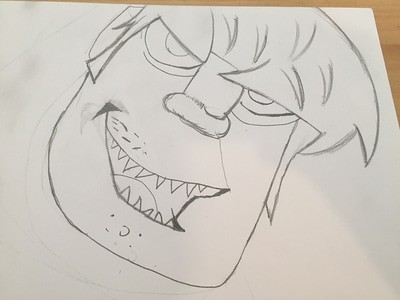This detailed pencil drawing on white paper showcases a close-up of an ogre's face, occupying most of the canvas. The ogre features a distinct square jawline and a wide, open-mouthed smile, revealing a pointed tongue and several sharp teeth on both the upper and lower jaws. A dimple graces the right side of his cheek, and whiskers are sketched above his upper lip and beneath his lower lip. His chin displays a pronounced cleft, adding to his rugged appearance. The eyes are simple circles with smaller circles inside, accentuated by wrinkles drawn underneath, giving a sense of depth and expression. The ogre's nose is stubby, complementing his overall fierce yet somewhat endearing look. Long strands of hair cascade halfway over his eyes, flanked by pronounced sideburns. A subtle light source illuminates parts of the paper, adding a gentle glow to the meticulous details of this fantastical creature.